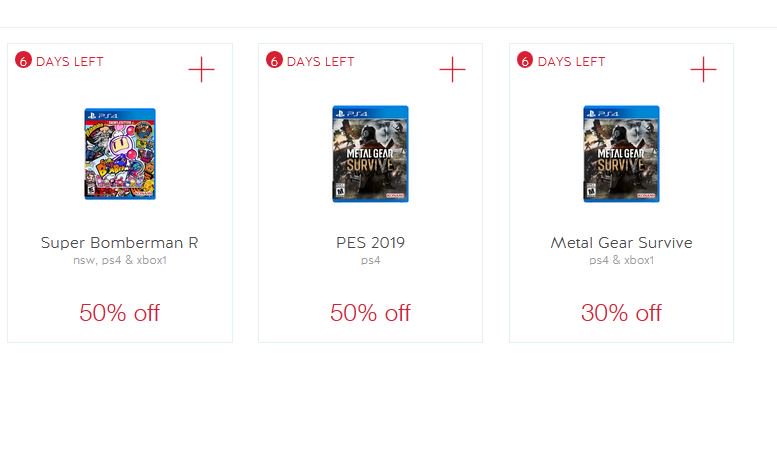The image showcases three PS4 game boxes arranged side-by-side, each enclosed in an outlined border of thin light gray lines, with a white interior. In the upper left corner of each box, there is a red circle with white font indicating the number of "Days Left" for the offer, placed next to the words "Days Left". A plus sign is situated in the upper right corner of each box. At the bottom center of each section, the discount percentage is prominently displayed: the first box offers 50% off, the second box also offers 50% off, and the third box offers 30% off.

The first game featured is "Super Bomberman R," displayed with a 50% discount. The middle box showcases "PES 2019," which offers a 50% discount and states "Metal Gear Survive" (although this may be an error in the image). The third box is correctly labeled "Metal Gear Survive" and presents a 30% discount.